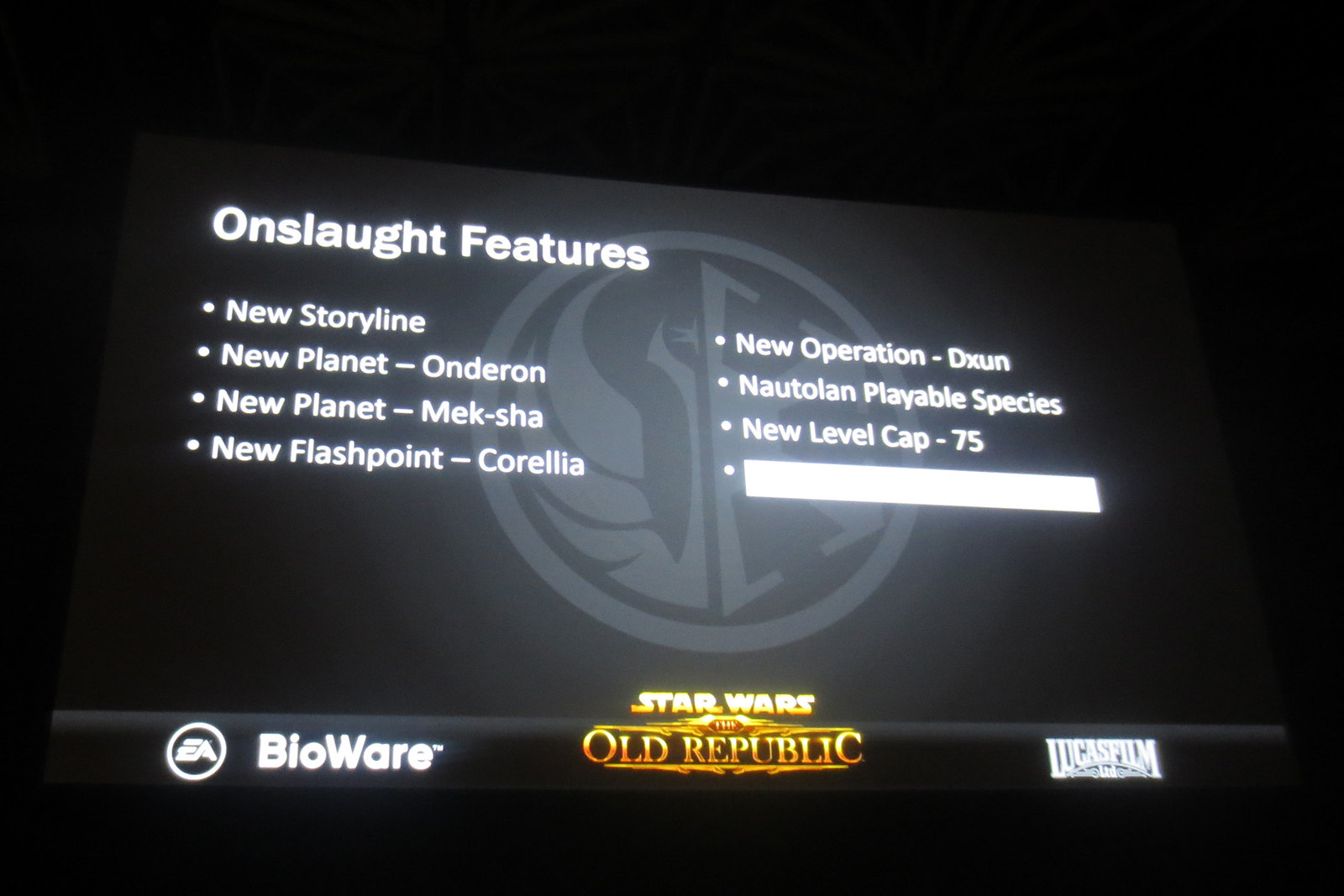The image captures a TV screen displaying the menu of "Star Wars: The Old Republic." The screen is in a dark room, with the monitor centrally positioned against a black background. The menu features the game’s logo prominently in the center, rendered in gold, along with the EA BioWare logo on the bottom left and the Lucasfilm Limited logo on the bottom right. In the background, there's a faint watermark of a Jedi logo. At the top of the screen, in white text, it reads "Onslaught Features" followed by a list of seven bullet points: "New Storyline," "New Planet: Onderon," "New Planet: Meksha," "New Flashpoint: Corellia," "New Operation: Dxun," "Nautolan Playable Species," and "New Level Cap: 75." The eighth bullet point is a blank white space. The overall color scheme of the image includes black, white, gray, yellow, red, and gold.